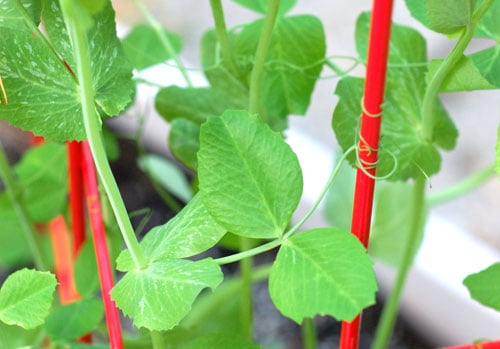In the image, we see a close-up, shallow-depth photograph of a vibrant green plant intertwined around red plastic support sticks. The bright green leaves, sprouting abundantly from vine-like stems, appear healthy and robust, showcasing the plant's lush vitality. The red plastic poles, used to support the plant, are clearly visible as they weave through the foliage. In the top left corner, one of the leaves exhibits small white markings. The background is slightly blurred, revealing a grayish soil or earth terrain and a white, possibly out-of-focus wall, suggesting the plants might be potted, although the details are indistinct. Additionally, a green cable or connector is vaguely discernible, intertwined with the plants. The photograph is taken in daylight, capturing the vivid colors and intricate details of the plants with a macro focus.